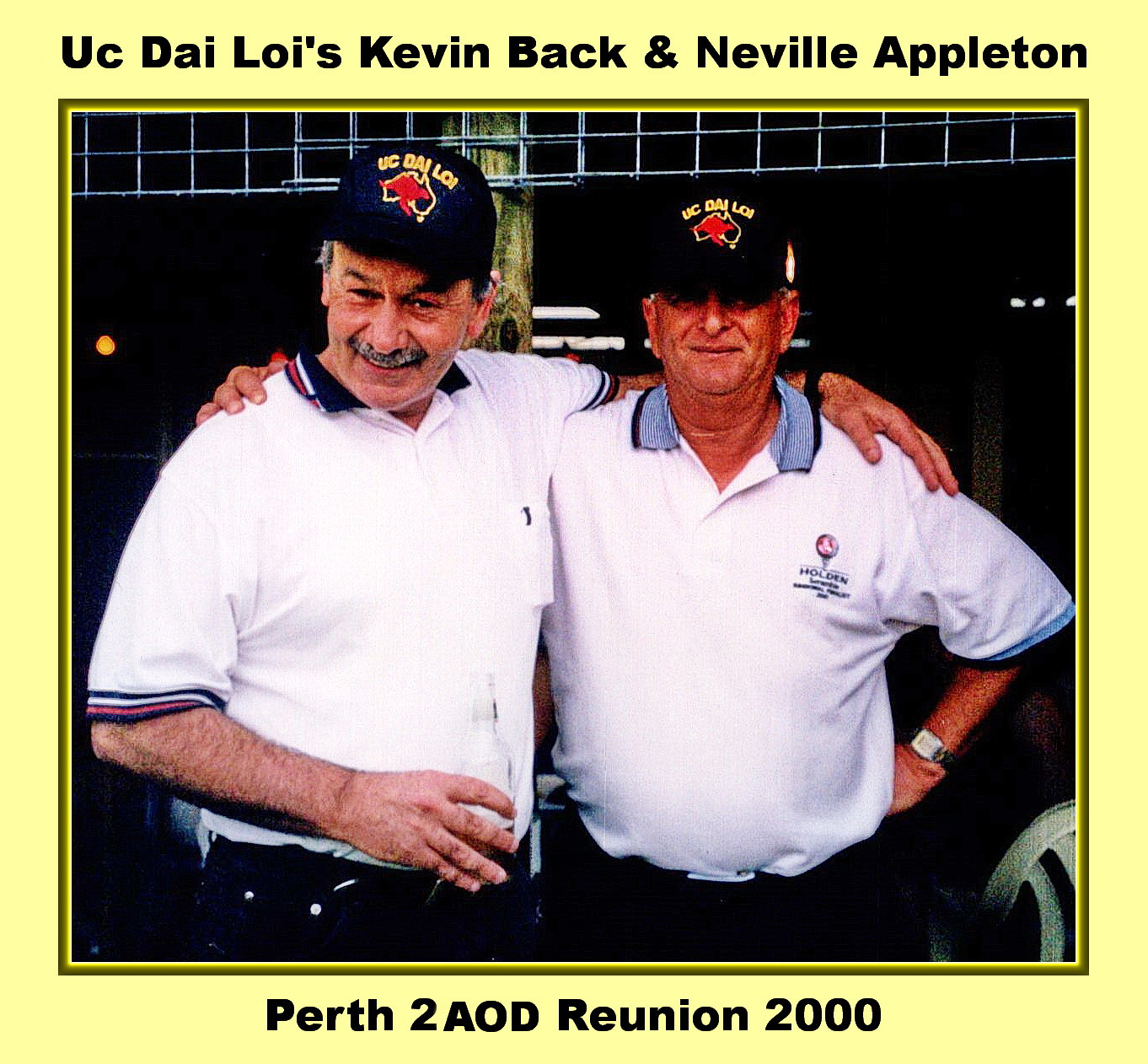This color photograph captures two older white men with their arms around each other, exuding camaraderie. Both are dressed in white polo shirts paired with black pants. Each man wears a black cap adorned with the text "UC DAI, Lewis," and a distinctive red and gold logo. The man on the left is holding a bottle, adding a casual touch to the photo. The background is very dark, though a crisscross metal bar, a pool, and a plastic chair are faintly visible. The photograph is framed with a white border, encased further by a yellow border with black text. At the top, the text reads "UC Dye, DAI, Lewis, Kevin Beck, and Neville Appleton," identifying the subjects. At the bottom, the inscription states "Perth, 2, AOD, Reunion 2000," indicating the location and event of the capture.